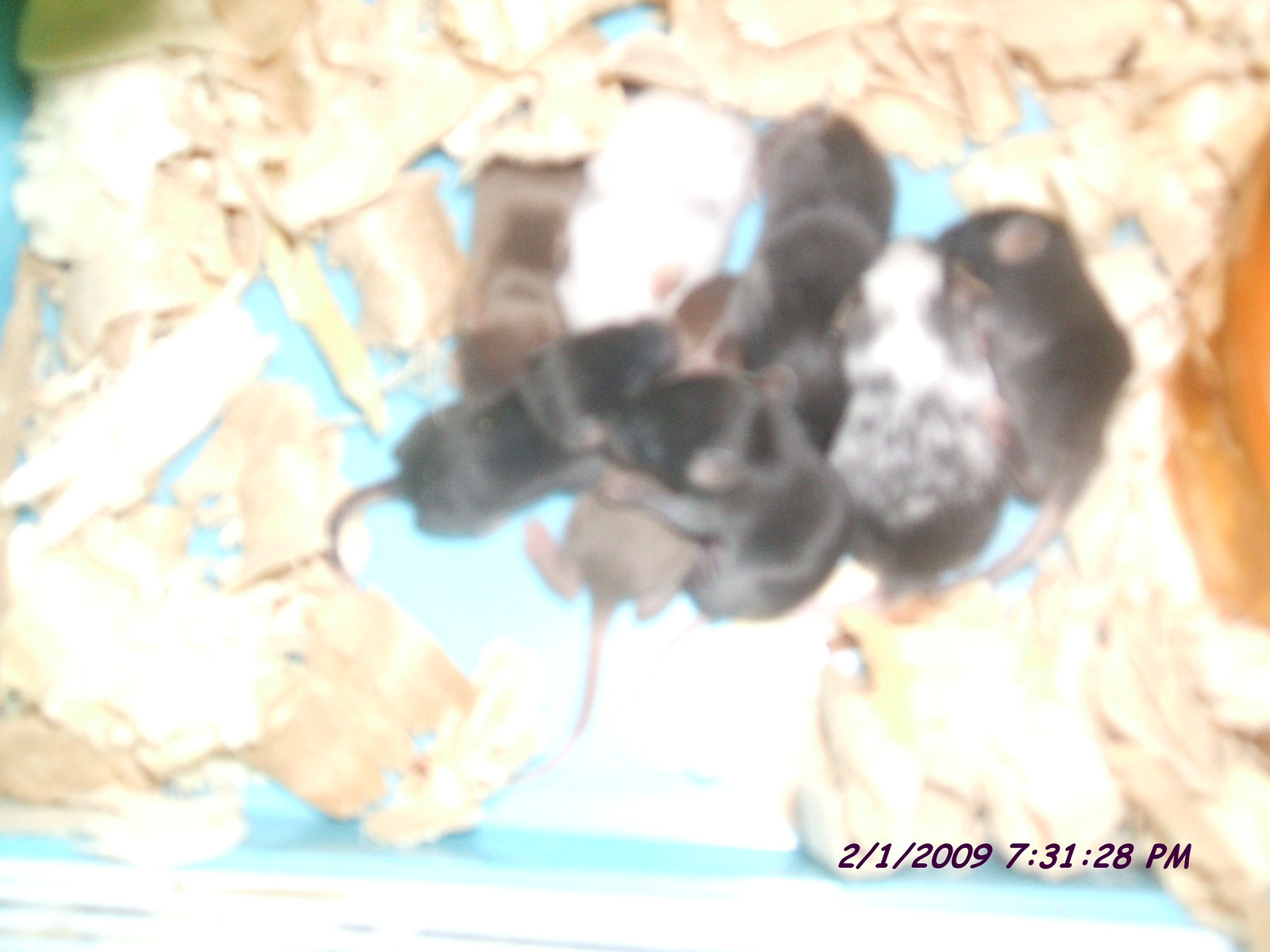This photograph, brightly lit but extremely blurry, depicts a group of newborn mice huddled together in a nest of shredded material—likely sawdust or insulation—on a light blue floor. The mice, some of which are black, white, and brown, form an indistinguishable mass due to the indistinctness of the image. Despite the blur, you can perceive their small, long tails and the fact that their eyes remain unopened. A time stamp in bold, dark purple text at the bottom right corner reads "2/1/2009 7:31:28 PM."